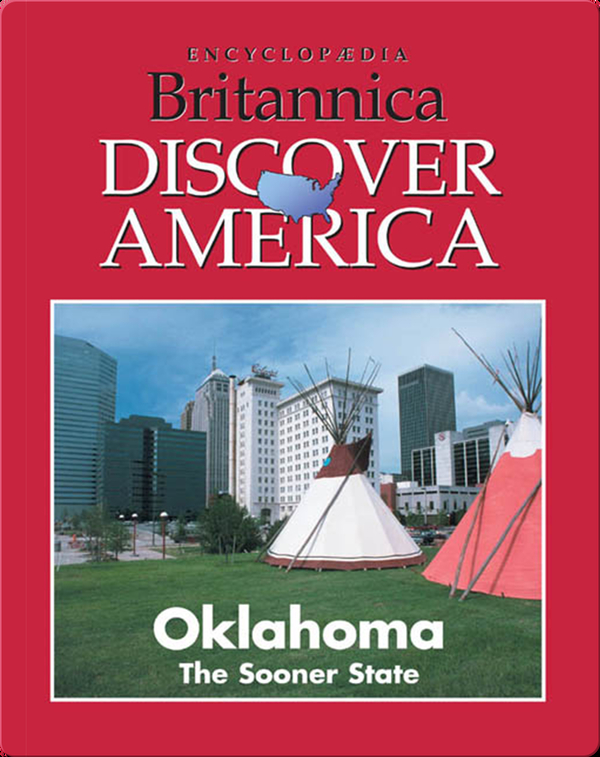The cover of the book is for Encyclopedia Britannica and prominently features the text "Encyclopedia Britannica Discover America" at the top in white letters, which includes a blue silhouette of the United States between the words "Discover" and "America." Below this, it reads "Oklahoma, the Sooner State" in white text. The background is a deep rosy red color, providing a striking contrast to the text and image.

The main image on the cover depicts two traditionally constructed teepees with stick poles, set on a lush green lawn in what appears to be a city park. One teepee is brown and white, while the other is a salmon color and white. Behind the teepees, the city's skyline is visible, including several high-rise buildings, trees, street lights, and a parking lot, indicating an unusual juxtaposition of traditional Native American structures within a modern urban setting. The book cover is a vertical rectangle, and the text is positioned horizontally. The overall style is evocative of an outdoor scene, tied together by the thematic elements of discovering America's diverse cultural and historical landscapes.